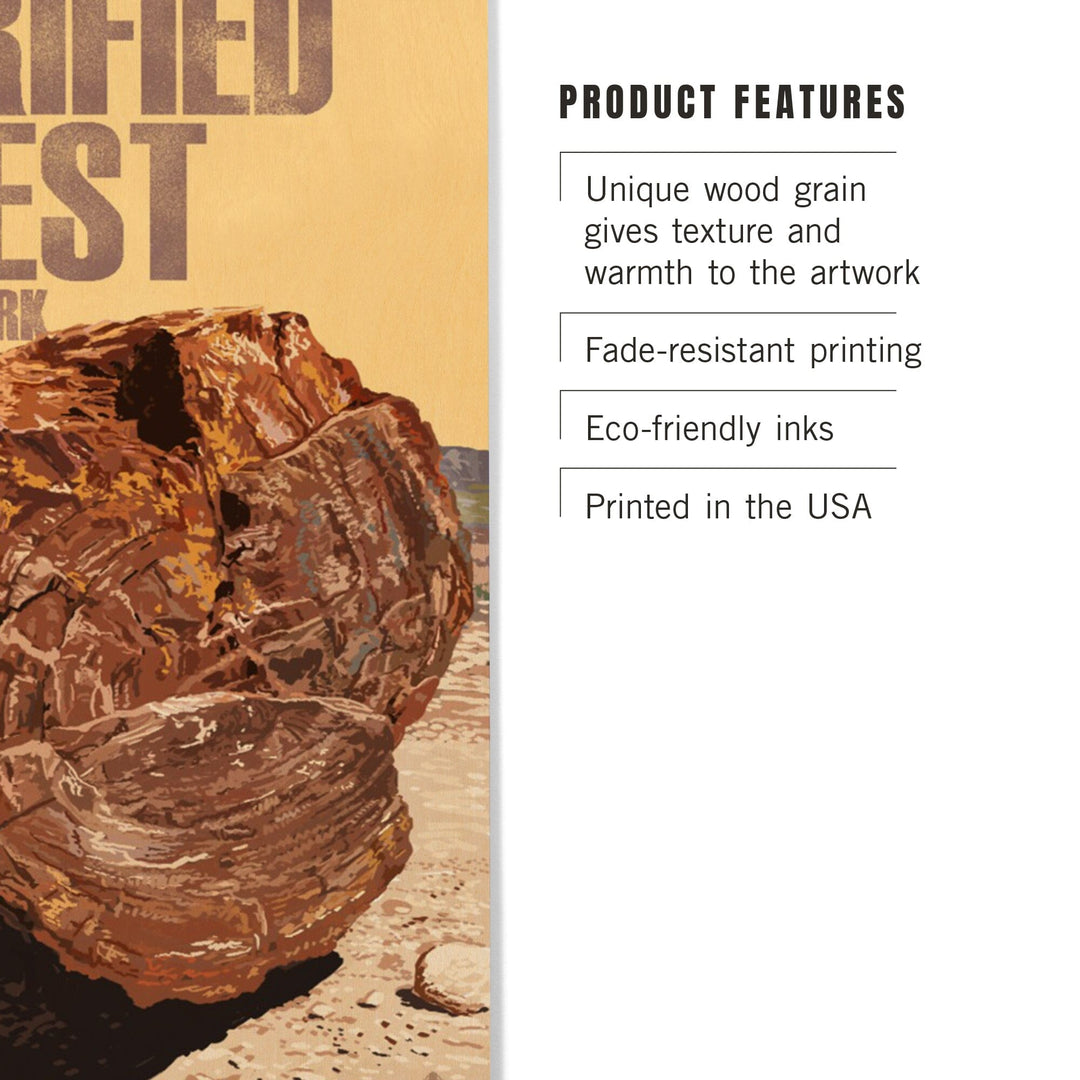The image is an advertisement for a wood-related product, featuring a painterly illustration on the left and descriptive text on the right. The illustration depicts a cut-down tree trunk with intricate details, showcasing unique wood grain. The trunk's interior displays an array of colors, including brown, black, beige, yellow, orange, and red, adding visual warmth and texture. The tree trunk sits on a light brown, rocky ground, casting a shadow, and the background transitions from a beige stone texture to green and blue tones with a mountain and field in the distance. Partially visible faded words in a brownish hue are present above the trunk. On the right, against a white background, are product features listed in black font: "Unique wood grain gives texture and warmth to the artwork," "Fade-resistant printing," "Eco-friendly inks," and "Printed in the USA."